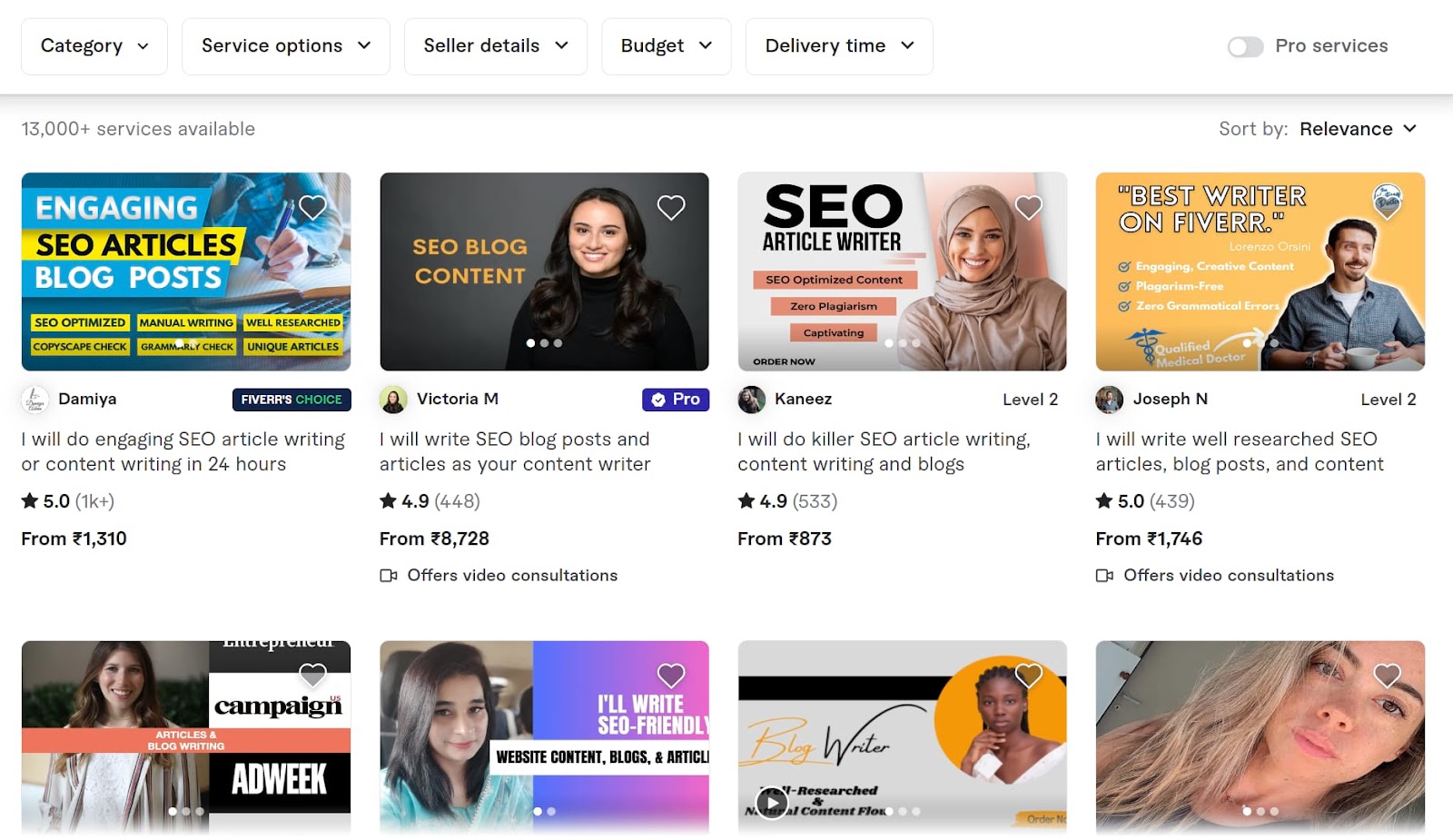Screenshot of a Website Description:

The screenshot depicts a section of a website featuring a series of options and service listings related to content writing and SEO services. At the top of the page, there are several filter boxes bordered by thin grey lines. These boxes are labeled "Category" with a down arrow, "Service Options" with a down arrow, "Seller Details" with a down arrow, "Budget" with a down arrow, and "Delivery Time" with a down arrow. 

In the top right corner, there is a toggle button for "WordPro Services." Below this segment, a line separates the filter options from the main content of the page. On the left side of this line, it states that over 13,000 services are available. To the right, the text reads "Sort by Relevance" with a down arrow. 

The main content area consists of eight boxes, each containing advertisements for different content writing services offered by various sellers:

1. The first box promotes a service for engaging in CEO articles and blog posts, with an image of a symbol and a small icon. The text offers to write CEO articles or content in 24 hours, boasting 5 stars from over 1,000 views out of 1,310 total. It also features an image of a woman smiling at the camera, branded as "Acterio M Pro," who offers to write CEO blog posts and articles with a rating of 4.9 stars from 448 reviews out of 8,728. This service includes video consultations.

2. Another listing under "CEO article writers" offers SEO articles with zero plagiarism under the name "Caffeine." This seller, "Knins," holds a Level Two status and has a 4.9-star rating from 533 ratings out of 873.

3. Promoted as the best writer on Fiverr, "Joseph N," also a Level Two seller, offers SEO articles, blog posts, and content writing services with a 5-star rating from 439 reviews out of 1,746. This service includes video consultations.

The bottom row showcases various writers, including images of women smiling:
- One writer, under the label "Word Campaign," offers articles and blog writing services.
- Another woman offers to write SEO-friendly website content, blogs, and articles.
- A third advertisement features a Black woman looking at the camera, branded as a blog writer.
- Lastly, there is another woman looking directly at the camera, with her service details not specified in the description.

This detailed layout provides comprehensive options for users seeking SEO articles, blog posts, and content writing services, complete with ratings, reviews, and additional service features like video consultations.